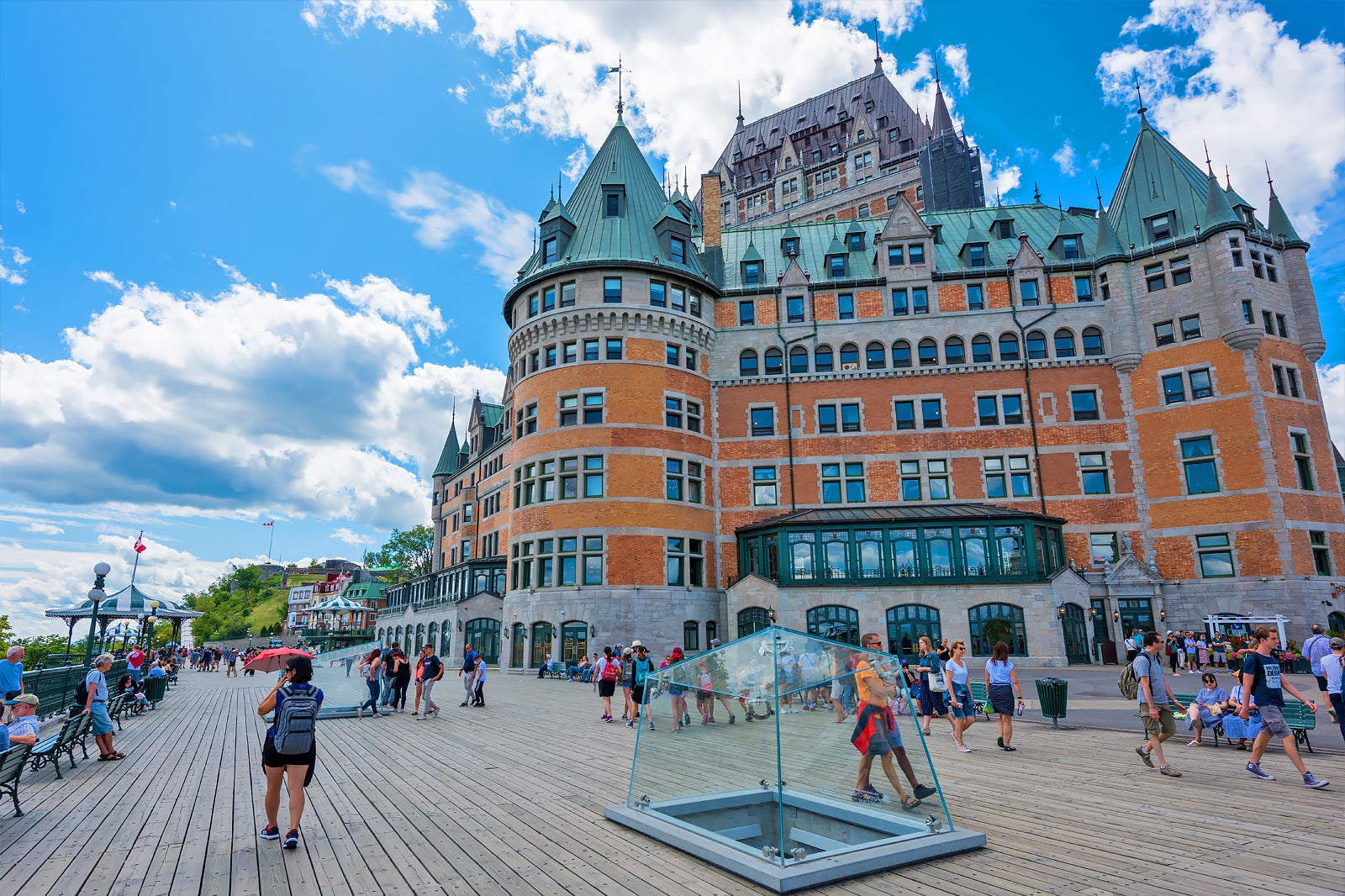In this bustling outdoor photograph, there is a prominent, enormous building featuring striking Germanic architecture. The structure, which spans multiple stories with a copper roof that has oxidized to green, stands tall with its distinctive orange-colored bricks. The facade transitions from a gray base to successive orange tiers, interspersed with numerous windows, and ends with a beige floor. This castle-like building boasts a vast wooden boardwalk in front of it, teeming with tourists. These visitors, dressed in summer attire such as shorts and t-shirts, wander about, capturing memories, lounging on benches, and strolling in groups. A noticeable skylight sits beside the edge of the image, adding a modern touch. To the left of the building, multiple trees and another large structure peek through, with a possible advertisement or billboard in the background. It's a sunny day, as evidenced by one lady’s red umbrella for shade and the overall lively, vibrant ambiance of a summer locale, possibly somewhere in Europe, like Germany or the UK. The vivid blue sky dotted with white clouds enhances the picturesque setting where this captivating scene unfolds.